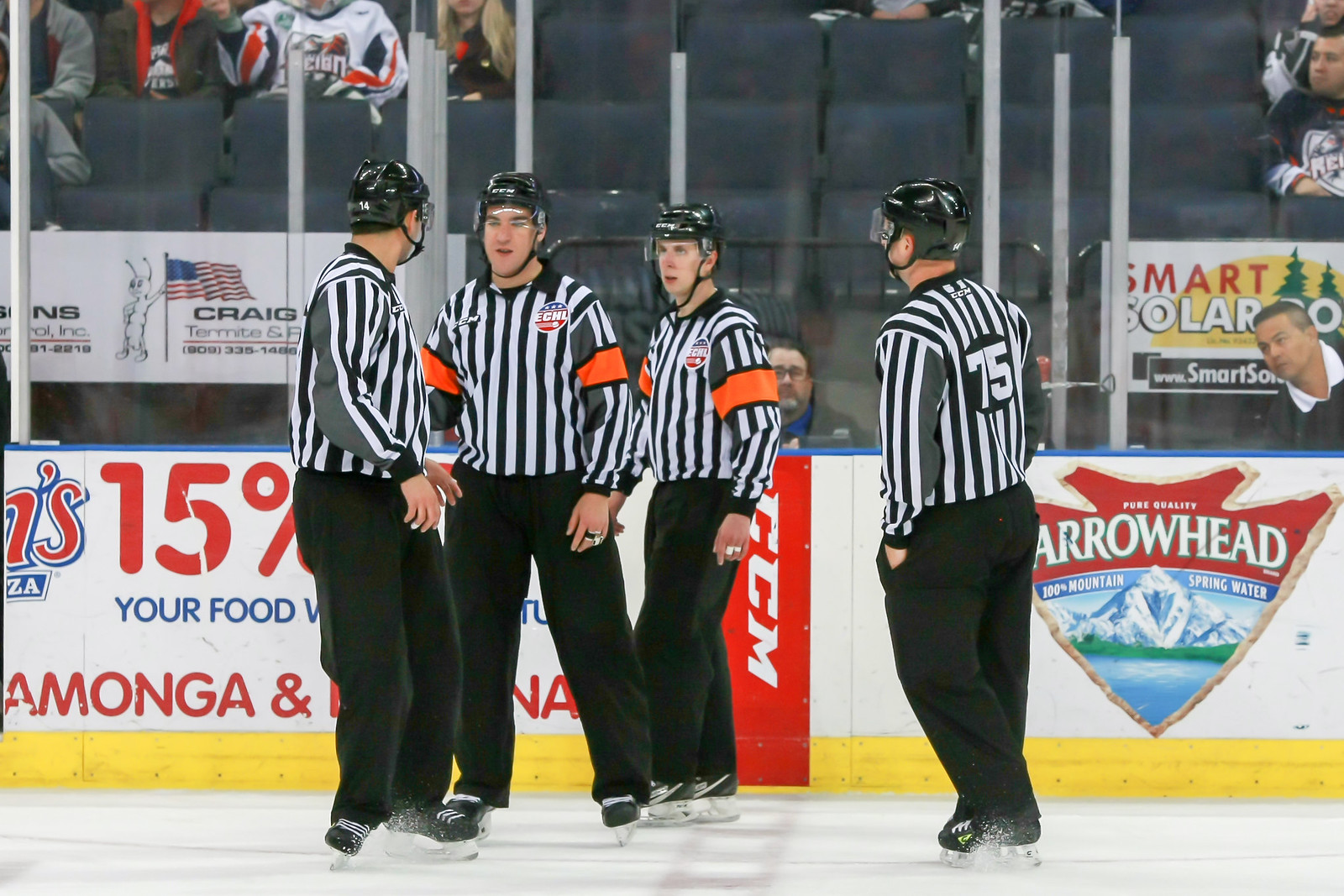This color photograph, taken inside an ice hockey rink, captures a close-up of four game officials huddled together in conversation on the ice. Each official is uniformly dressed in black helmets with transparent visors, black and white striped long-sleeve shirts, and black pants. They all wear black leather ice skates with silver blades. The background reveals a plexiglass barrier separating the rink from the stands. While most of the seats behind them are empty, a few spectators are visible seated further away. An advertisement for Arrowhead Water is prominent behind the referee on the far right, and an American flag can be seen in the distance. The rink also features additional advertisement borders, including some related to food.